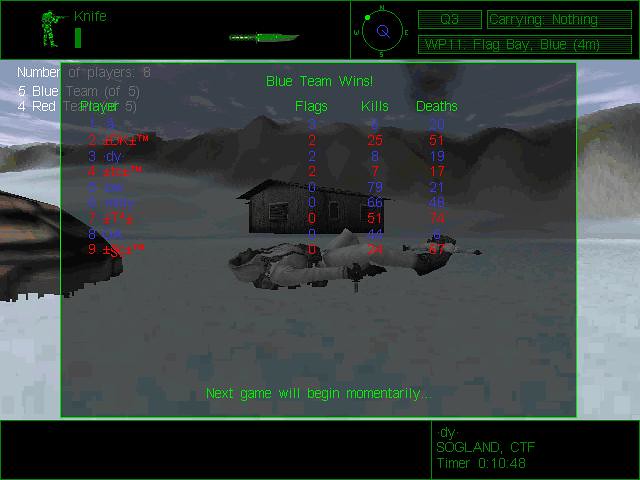This is a screenshot from a video game depicting a poignant winter scene, highlighted by a somber atmosphere and dire conclusion. The background showcases the main character, clad entirely in a white snowsuit, lying lifelessly on their back with limbs splayed, gazing blankly upward. The translucent gray overlay denotes the game's conclusion, allowing a faint view of the fallen hero beneath it. 

Emblazoned across the center in green script is the triumphant message "Blue Team Wins," accompanied by detailed player statistics featuring categories like flags, kills, and deaths, presented in vibrant red and deep blue tones. The footer displays the final scores and cheerfully informs, in vivid green, "Next game will begin momentarily."

In the top-left corner, a small character icon reveals the protagonist's last known possession - a knife - while the top-right side likely displays a map and weapon status, noting the character is currently unarmed. Additional game details are noted along the bottom, including the cryptic "DY, slow gland, CTF," and a timer reading 01:04:48. This image captures the essence of a climactic and somber end-game moment framed within an icy, digital battlefield.